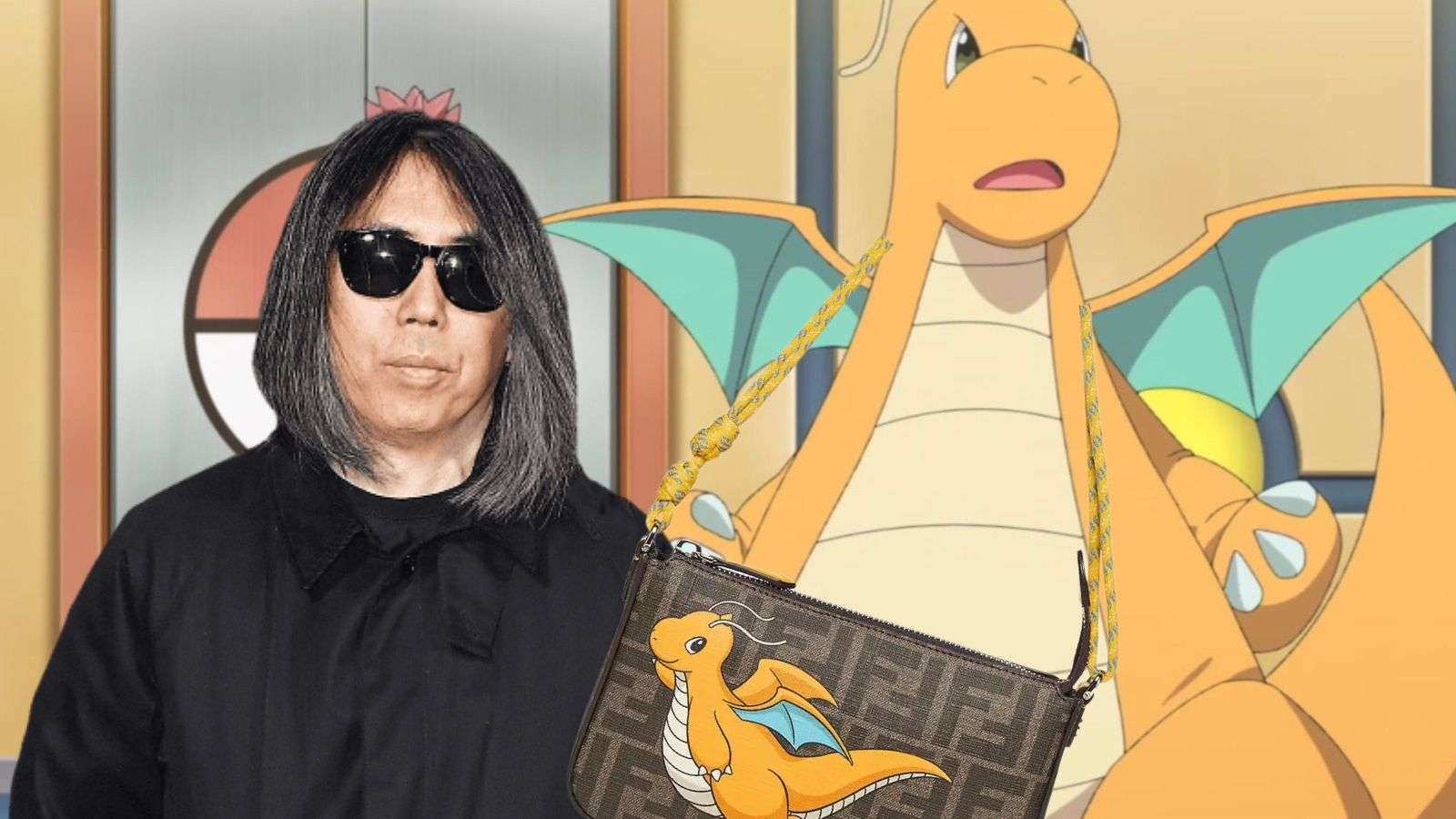This photograph features an Asian woman standing to the left, wearing black glasses, a black button-down shirt, and a black shirt underneath. She is holding a brown purse adorned with an upscale pattern of the letter 'F', both upright and upside down. The purse has a distinctive yellow and blue roped handle and prominently displays an orange dragon-like Pokémon, resembling Charizard, characterized by its blue under-wing coloring, white-striped belly, and three claws on each paw. In the background, partially obscured by the woman's head, there is a silver elevator door with a visible line down its center and what appears to be a Pokéball. To the right side of the image, a larger depiction of Charizard is visible, showcasing its white belly, orange wings with blue undersides, and outstretched arms, looking off to the left.